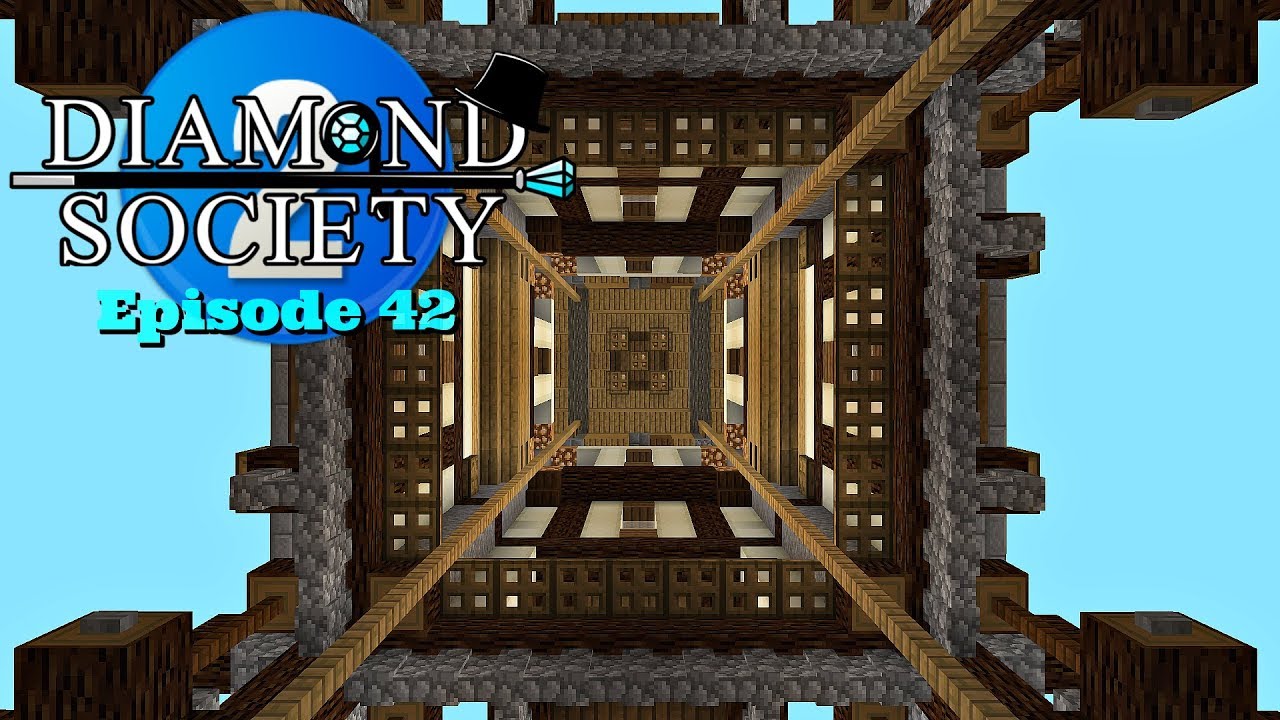The image appears to be a computer-generated, rectangular depiction reminiscent of an old-school video game, possibly Minecraft. It is primarily composed in a landscape layout, where the top and bottom edges are longer than the sides. The background is a bright, baby blue color. In the upper left corner, there is a round blue circle with a white number two. Overlaying this circle are the words "Diamond Society" in white lettering and "Episode 42" in blue text. The main focus of the image seems to be a view looking either up or down a passageway or an elevator shaft, constructed with block-like features in shades of brown and gray. The perspective reveals a tall, intricate, three-dimensional design, possibly mimicking stone and wood patterns. The bottom of the image features solid brown panels lined with gray striping, and in the center are five squares with varying patterns and textures, contributing to the overall video game aesthetic. The corners of the image contain additional square wood shapes, enhancing the geometric feel.